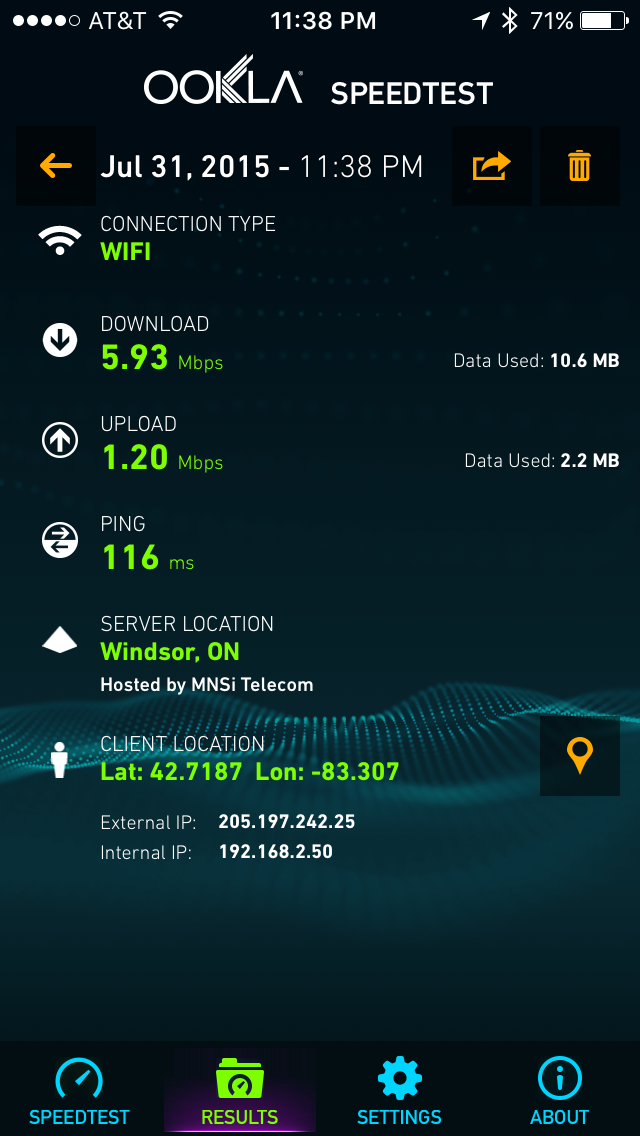This image is a detailed screenshot of a mobile device displaying the Ookla Speedtest app interface. At the top, the notification bar shows various icons including AT&T with a signal symbol, the time, 11:38 PM, and a battery icon at 71%. Below this, prominently in the center, the app details are displayed in white text: "Ookla Speed Test, July 31st, 2015, 11:38 PM." The results indicate a connection type of WiFi with a download speed of 5.93 Mbps, an upload speed of 1.20 Mbps, and a ping of 116 ms. The server location is Windsor ON, hosted by MNSI Telecom, and the client location is specified as Lat 42.7187, Long -83.307 with an External IP 205.197.242.25 and Internal IP 192.168.2.50. The background features a wavy pattern in blue hues and a dark blue backdrop. At the bottom of the screen, there are four icons labeled "Speedtest," "Results," "Settings," and "About." The overall theme includes colors of white, black, turquoise, and orange, and the image gives an impression of a structured and data-rich interface typical of an iOS app.